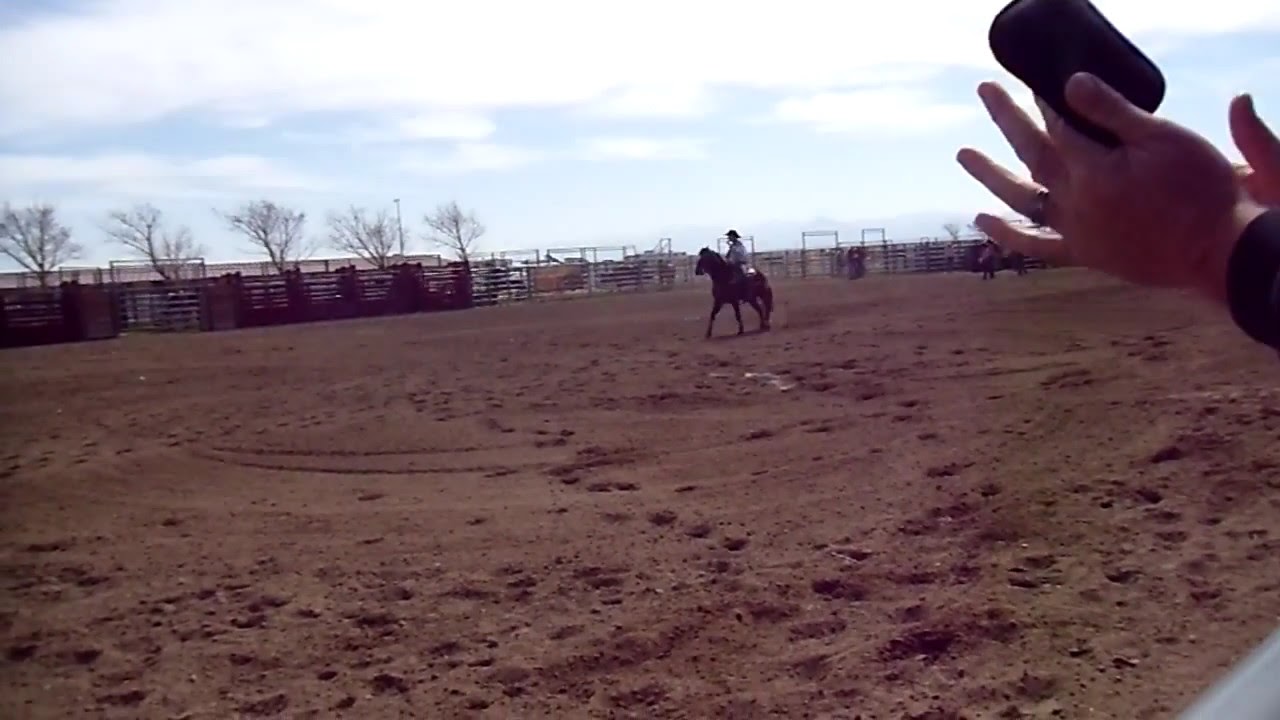The image depicts a sprawling, flat field of tan and brown dirt, reminiscent of a rodeo arena, with scattered hoof prints creating a textured, moon-like surface. In the middle of the field, a person sits astride a small brown horse, their attire suggesting a cowboy-like figure with a black hat and a white shirt. The area is enclosed by a mix of wooden and metal fencing, and leafless trees can be seen lining the fence on the left. Overhead, thin clouds drift across a pale, whitish-blue sky, contrasting with the dimly lit ground. On the right side of the image, a pair of hands with a wedding ring and a small black object are held up, possibly clapping, creating a sense of engagement and movement in the otherwise distant and serene scene.